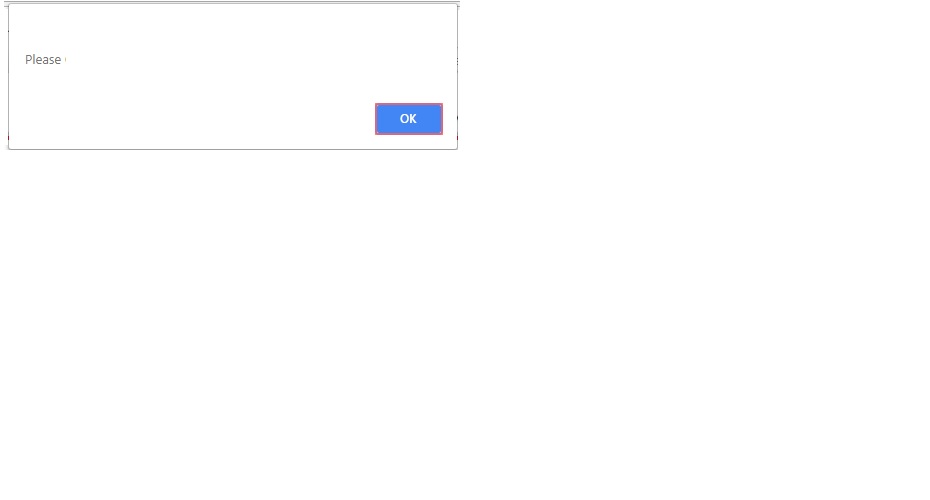The image features a simple horizontal rectangle with a white background, defined by a gray outline. The rectangle itself is white, differentiated from the background only by this border. Positioned to the left within the rectangle is the word "Please," written in small, gray letters with a capital "P." 

On the lower right corner inside the rectangle, there is a button designed to resemble a clickable or tappable interface element. This button is a small blue rectangle outlined in red, containing the text "OK" in white, capital letters. Additionally, the gray outline of the main rectangle shows minor imperfections, with tiny red dots visible in three locations: two on the right side and one on the left.